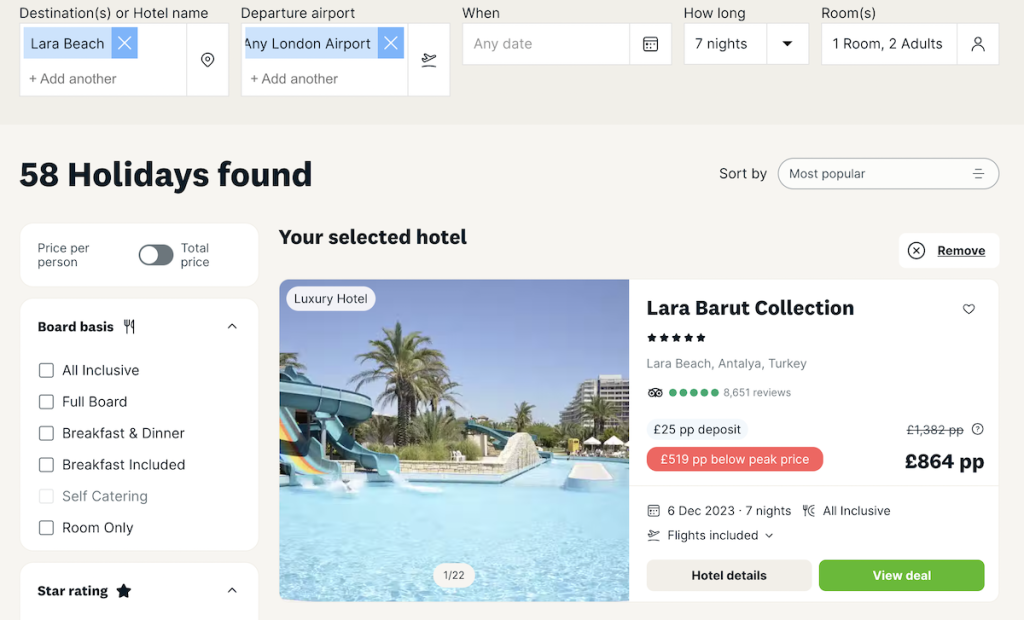The image depicts a travel booking website search page dedicated to selecting a holiday destination. At the top of the page, there are search fields labeled "Destinations or Hotel Name," "Departure Airport," "When," "How Long," and "Rooms." The user has input "Laura Beach" under the destination, "Any London airport" as the departure point, selected a duration of seven nights, and specified the search for one room for two adults. Below these search parameters, the website displays the results, indicating that 58 holiday options have been found. 

Prominently featured is a listing for the "Laura Barut Collection," a luxurious hotel. The listing includes an image showcasing the hotel's amenities, such as a swimming pool flanked by palm trees, and water slides. The hotel has received a five-star rating. The total price for the stay is listed at £864 per person (indicated by "PP"). The listing notes that there have been numerous positive ratings and mentions a required deposit of £25.